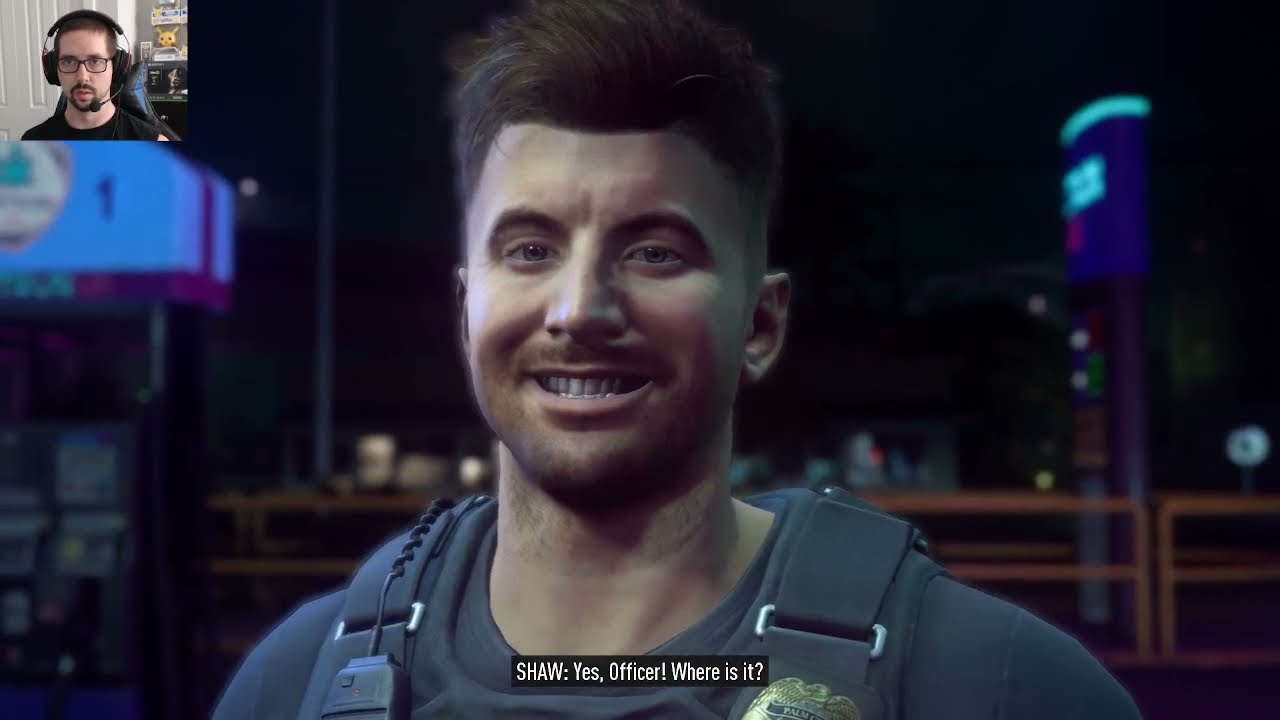The image depicts a streaming session featuring a live video game. In the upper left corner, there is a small window showing the streamer. The streamer has short brown hair, glasses, a black gaming headset, and a black t-shirt, sitting on a gaming chair with a shelf and a white door in the background. The main portion of the image is a computer-generated screenshot of a video game featuring a Caucasian police officer with brown hair, thick eyebrows, a beard, and a mustache. The officer is smiling, dressed in a bulletproof vest with a police badge and a walkie-talkie attached. The game environment appears to be a cityscape at night, with a yellow and pink railing visible in the background. Subtitles at the bottom of the image read, "Yes, officer! Where is it?" indicating in-game dialogue. The combined setup highlights the streamer’s engagement with the game and the real-time interaction unfolding onscreen.